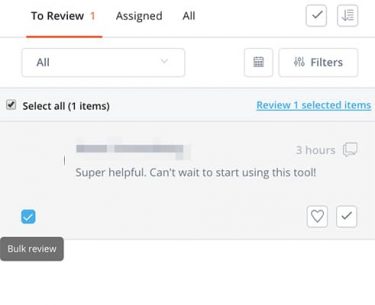The image appears to depict a user interface for a review or task management tool. At the top, there is a header section that includes a red-highlighted, underlined “Review 1” prompt, followed by a drop-down menu option labeled "All." To the right of this menu, there are two adjacent squares - one black and one white with gray edging. Next to these squares is a "Filters" button.

Below this header section, there's another rectangular area featuring a button or a checkmark labeled "Select all 1 item" on the left, and on the far right, the text "Review 1 selected item" appears in blue and underlined.

In the main content area beneath this, there is an item that has been grayed out. A comment left by a user reads: "Super helpful, can't wait to start using this tool" from three hours ago. This comment is accompanied by a checkmark in a white box and a heart in a white box on the bottom right.

Further down, there is a gray button labeled "Bulk Review" on the bottom left, next to a checkmark in a blue box. At the upper right corner of the interface, there is a checkbox in a white box and an icon resembling a downward-pointing arrow within a box that has horizontal lines.

This caption offers a comprehensive description of the various elements and layout found in the user interface of the tool.